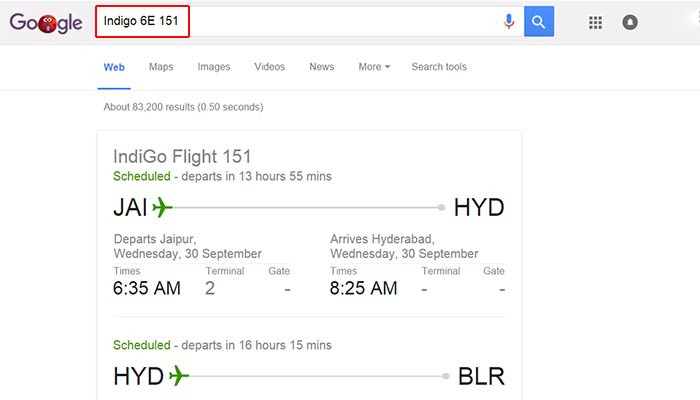This is a detailed screenshot of a Google search results page. In the top left corner, the Google logo is creatively altered, with a red M&M character replacing the second "O" in "Google," showcasing one of Google’s playful, temporary art logos. In the search bar, the text "IndiGo SE 151" has been entered and is outlined in a red box. To the right side of the search bar, there are two icons: a blue and red microphone for voice search and a blue box with a white magnifying glass for initiating a search.

Below the search bar, there are various filter options available, each labeled as: Web, Maps, Images, Videos, News, More, and Search Tools. The "Web" filter is highlighted in blue and underlined, indicating the current selection. Beneath these filters, prominent flight information for "IndiGo Flight 151" is displayed within a white square. The details indicate that the flight is scheduled, highlighted in green, and is set to depart in 13 hours and 55 minutes.